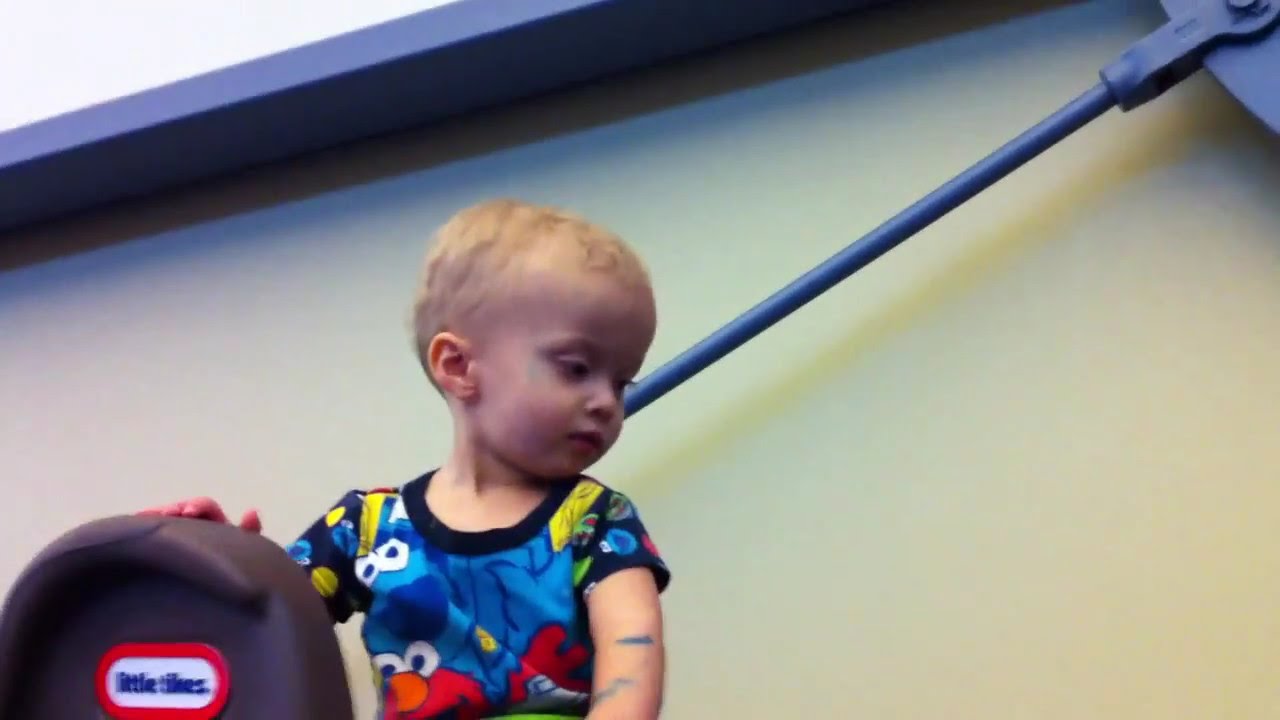This detailed photograph captures a child, likely around one and a half to two years old, with sparse light blonde hair, seen from a side angle looking down to the lower right. The child is wearing a short-sleeved top featuring Sesame Street characters, prominently including Elmo on an ocean blue background, possibly resembling pajamas with blue, yellow, red, and white colors. Their right hand rests on a dark brown plastic molded object, partially visible with a distinguishable "Little Tikes" logo in navy and ocean blue print on a white background with red trim, suggesting it might be a toy motorbike or another riding toy. The background of the image reveals a yellow backdrop with a blue metal bar leading to a brace and round piece in the upper right corner, alongside a blue ledge and overhang, contributing to an overall playful and childlike scene.